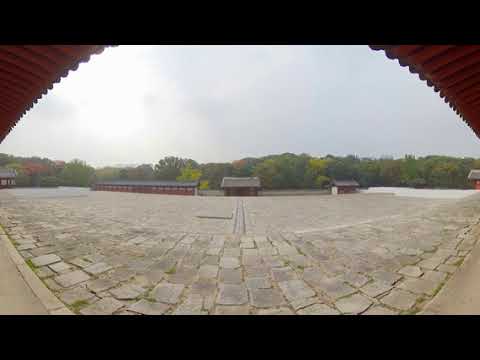The image showcases an outdoor scene in a small, rural Asian town, viewed through a fisheye lens at a slight angle. To the left, there is a long red building with a gray-ish black tiled roof, reminiscent of traditional Asian farm buildings seen in historic settings. The paved area or courtyard in the foreground is composed of mostly square but somewhat rectangular stone masonry, with grass sprouting up between the pavers. This courtyard is vast and spacious, evoking the setting of movie scenes where generals meet with their soldiers. In the distant center, a cluster of small buildings can be seen, with a dense tree line forming the backdrop. The perspective is from underneath a corrugated roof, possibly of a similar architectural style. The scene is set during the daytime with overcast skies, giving an impression of an imminent rain, and there are no shadows present to indicate the time of day.